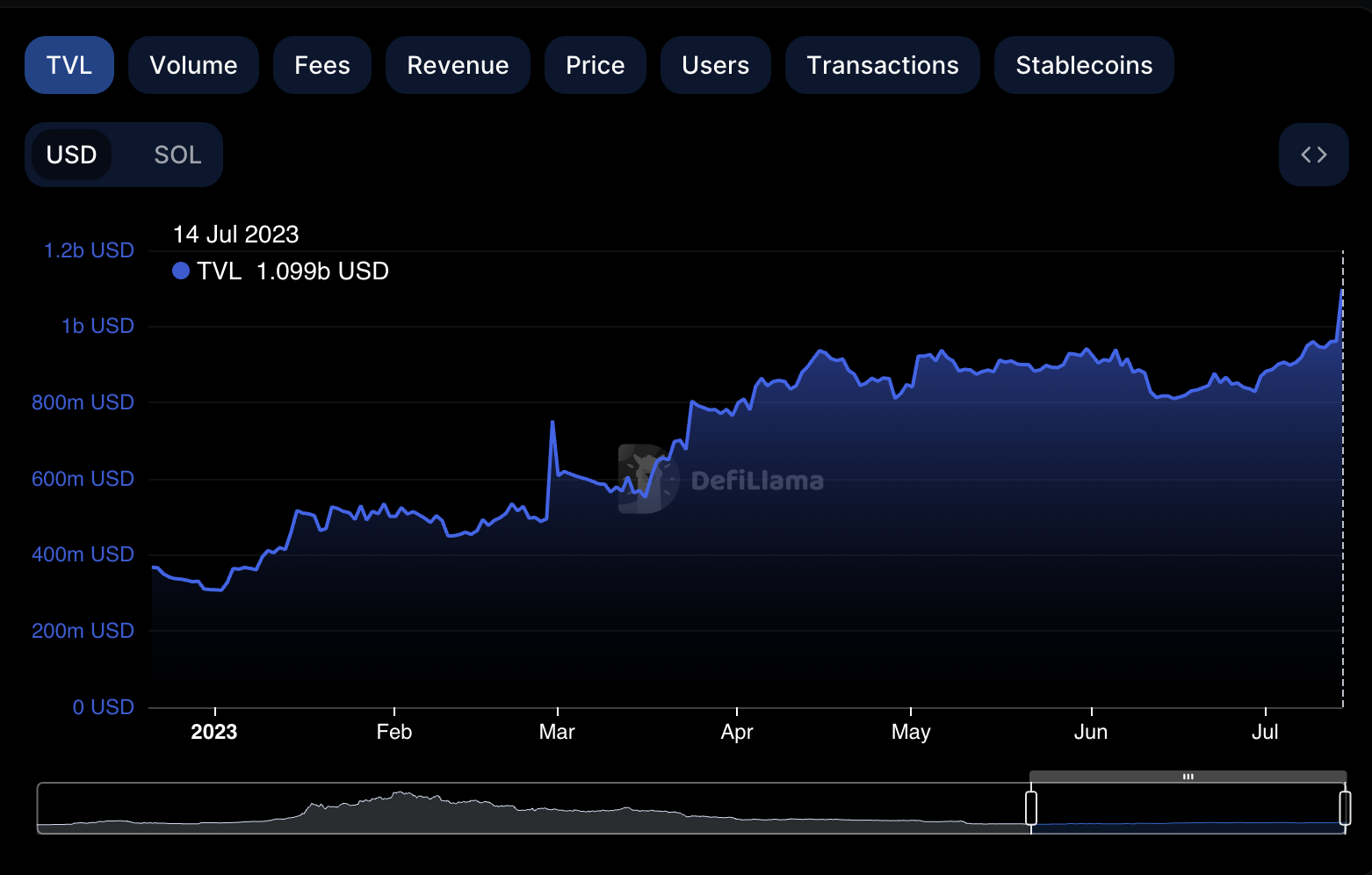The image presents a comprehensive graph primarily focused on cryptocurrency metrics, depicted on a dark background. The heading "TVL" (Total Value Locked) stands out in vibrant blue text, indicating the primary data being visualized. Other metrics such as "Volume," "Fees," "Revenue," "Price," "Users," "Transactions," and "Stable Coins" are labeled in white text, encased in faint, nearly invisible boxes that can be highlighted by selection, similar to the highlighted "TVL."

Positioned next to "USD," which is highlighted, is "SOL." The left vertical axis enumerates values starting from 0 USD and incrementing by 200 million USD up to 1.2 billion USD. Near the top, adjacent to the 1.2 billion USD mark, is a blue dot, conspicuously bright, that points to a value on 14 July 2023: TVL at 1.099 billion USD.

The horizontal axis at the bottom charts time from February 2023 to July 2023, marked with equidistant labels for each month. A vertical dashed line runs along the right side, and above it, there are "<" and ">" symbols.

Additionally, a secondary smaller graph lies beneath, featuring a timeline with peaks and troughs delineated by slider bars. This smaller graph starts flat, rises to a peak, and then gradually declines. The active slider ranges from around June to the end of July 2023, capturing a segment of the timeline.